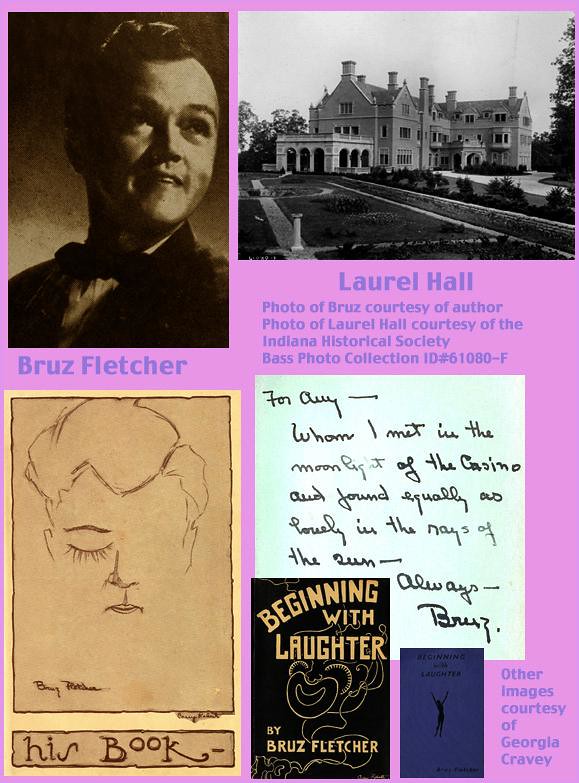This image depicts a collage-style page, likely from a scrapbook or a memorial poster, set against a vibrant pink background. In the top left corner, there is a vintage black-and-white photograph of a clean-shaven man with short-cropped hair, identified as Bruz Fletcher. Beneath his picture, in purple font, it says "Bruz Fletcher." Adjacent to his photo is an artistic rendering featuring a stylized half-sketch of a face with an eye, nose, and lips, and the words "his book" in brown font below it.

To the right side of the collage, there is a black-and-white photograph of an elaborate mansion identified as Laurel Hall, with multiple gables and a three-story structure giving it a majestic appearance. Underneath, a caption states "Photo of Laurel Hall, courtesy of the Indiana Historical Society," along with "Bass Photo Collection ID number 61080-F."

Interspersed among the images are handwritten notes and literary cutouts, adding to the collage's vintage aesthetic. Notably, there's a handwritten note saying, "for whom I met in the moonlight of the casino and found equally as lovely in the rays of the sun. Always Bruce."

In the lower portion of the collage are miniatures of book covers by Bruce Fletcher, including one titled "Beginning with Laughter," featuring a pointillistic-style image of a clown on a black background. The page is sprinkled with other elements, such as more handwritten notes and images, credited "Other Images Courtesy of Georgia Cravey." The various hues of purple, black, white, gray, and dark blue contribute to the nostalgic and commemorative tone of the page, celebrating the life and works of Bruz Fletcher.